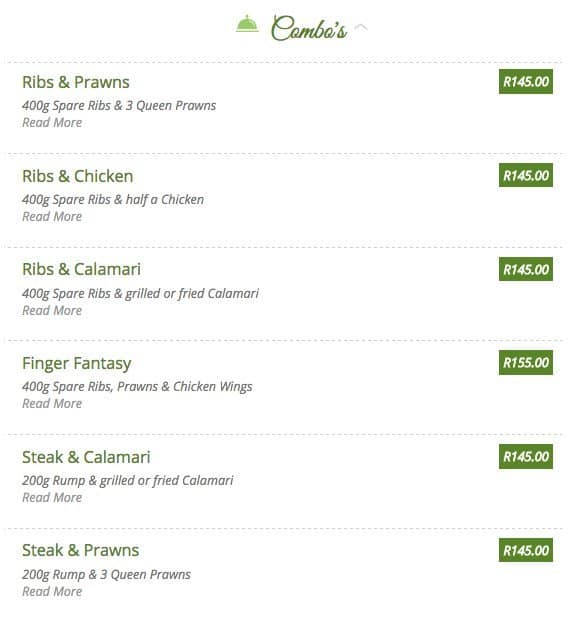This image is a screenshot of a restaurant menu, specifically displaying various food combos. At the top of the menu, there is an illustration of a cloche, the classic domed cover that chefs use to present dishes. The section header is titled "Combos," written in green font.

The menu lists the following combo options, along with their details and prices:

1. **Ribs and Prawns**: 400g spare ribs accompanied by 3 queen prawns, priced at R145.
2. **Ribs and Chicken**: The cost for this option is also R145.
3. **Ribs and Calamari**: Available for R145.
4. **Finger Fantasy**: A combination of spare ribs, prawns, and chicken wings, priced at R155.
5. **Steak and Calamari**: Available for R155.
6. **Steak and Prawns**: This includes a 200g rump steak and 3 queen prawns, priced at R145.

The menu options mostly feature uniform pricing, with a few exceptions noted for more expansive combinations.